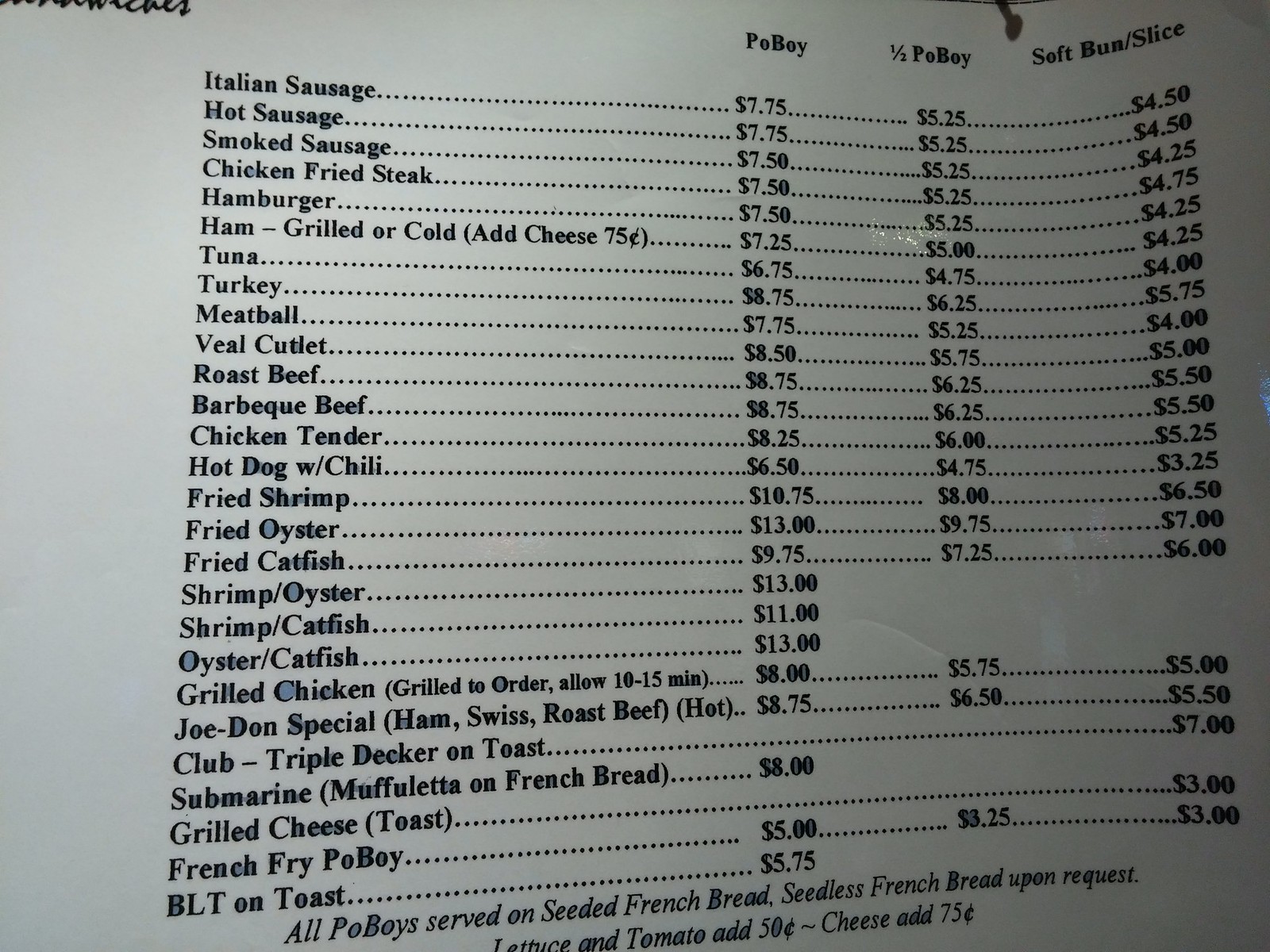Here is a detailed and cleaned-up caption for the described image:

---

Image Description: A menu sheet for sandwiches, featuring a variety of options with corresponding prices indicated by dotted lines. The menu, printed on standard paper, has some obscured writing in the upper left-hand corner. It offers multiple preparation styles for each sandwich: as a po' boy, a half po' boy, or on a soft bun/slice. The list of sandwich options is extensive, including Italian sausage, hot sausage, smoked sausage, chicken fried steak, hamburger, ham (grilled or cold, with an option to add cheese for 75 cents), tuna, turkey, meatball, veal cutlet, roast beef, barbecue beef, chicken tenders, hot dog with chili, fried shrimp, fried oyster, fried catfish, shrimp & oyster, shrimp & catfish, oyster & catfish, grilled chicken (prepared to order, with a 10 to 15-minute wait time), Joe Don special (ham, Swiss, roast beef, served hot), club (triple decker on toast), submarine, mufalada on French bread, grilled cheese, toast, French fry po' boy, and BLT on toast. All po' boys are served on seeded French bread, with seedless French bread available upon request, and additional toppings like lettuce and tomato for 50 cents and cheese for 75 cents. Notably, the menu paper has been marked by a reportedly bored customer, who filled in many of the O's and D's along with some other letters using a pencil, perhaps to pass the time.

---